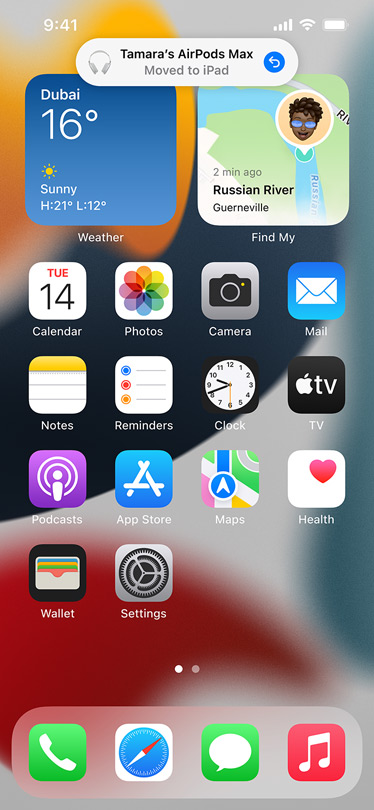This photograph captures the front homepage of a cell phone. The background of the screen features a blurred, abstract image with a gradient of colors: yellow at the top, transitioning to black or dark navy in the middle, and finally to red at the bottom, with a touch of white mixed in.

At the top of the screen, there's an icon representing headphones with the label "Tamera's AirPods Max," accompanied by an option to "Move to iPad." A blue button with a circular arrow is also visible in this section.

Just below, the weather information is prominently displayed: "Dubai, 16 degrees, sunny," followed by a forecast indicating a high of 21 degrees and a low of 12 degrees. To the right of the weather details, there is a recent activity notification that states, "two minutes ago, Russian River, Guantanamo," accompanied by an avatar. This avatar is a cartoon depiction of an African-American person with black hair and sunglasses.

Further down, the screen displays a grid of various app icons, including Calendar, Photos, Camera, Mail, Notes, Reminders, Clock, and TV, among others, showcasing the user's diverse app collection.